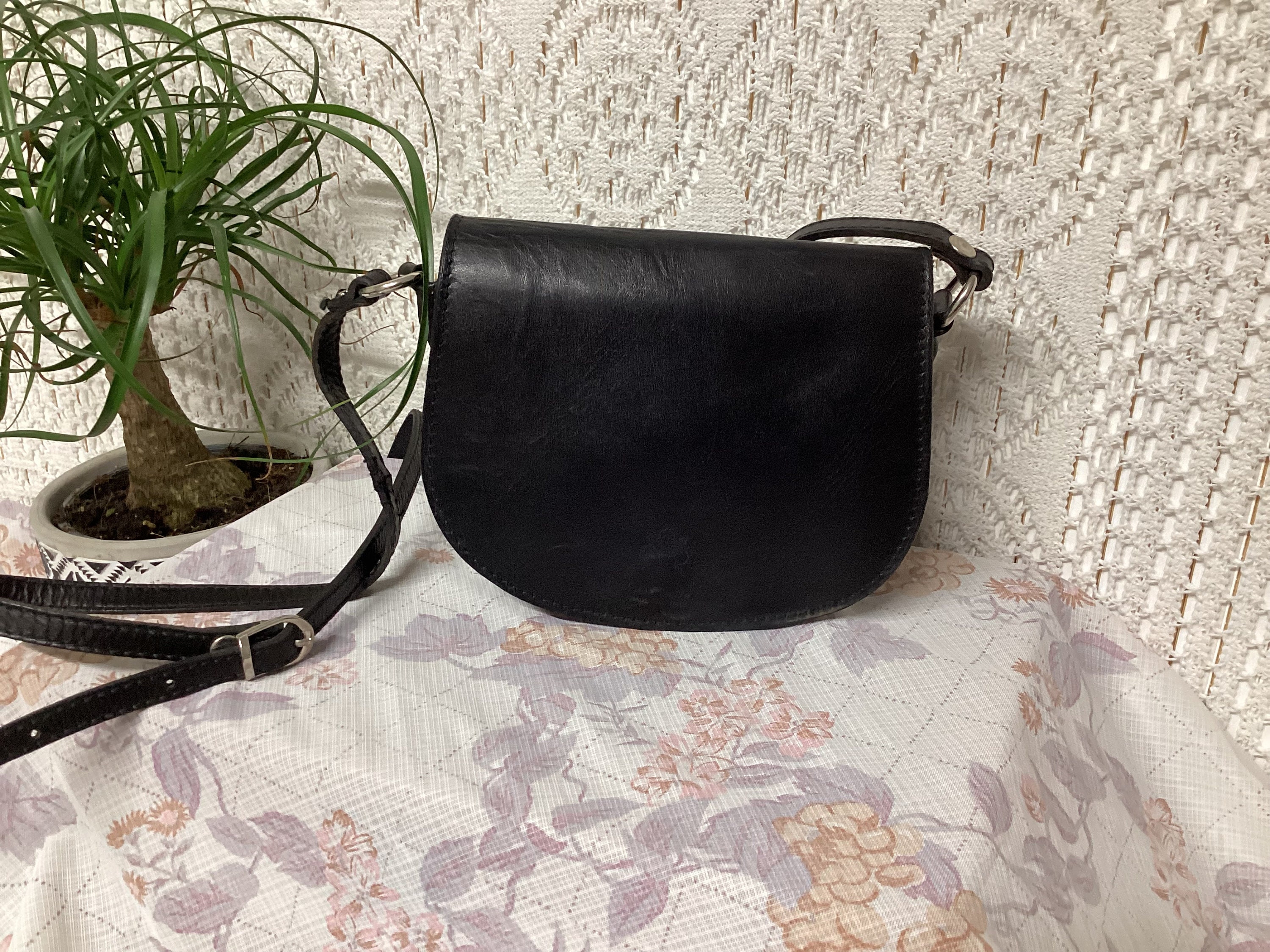The image features a black leather purse with a silver buckle on its adjustable strap, prominently placed on a table covered with a floral-patterned fabric. The fabric showcases a mix of colors including dark gray, yellow-red flowers, and pink and purple motifs. Right beside the purse, to its left, there's a potted plant in a thick, painted clay pot. The pot has black and white hues, which adds to the visual interest with its striking greenery spilling out. In the background, a manufactured crochet or macrame wall hanging in beige, featuring circular and diamond patterns, adds a textured backdrop to the scene. The overall color palette consists of black, white, gray, yellow, tans, and subtle hints of pink and purple, contributing to a balanced, though slightly eclectic, composition.